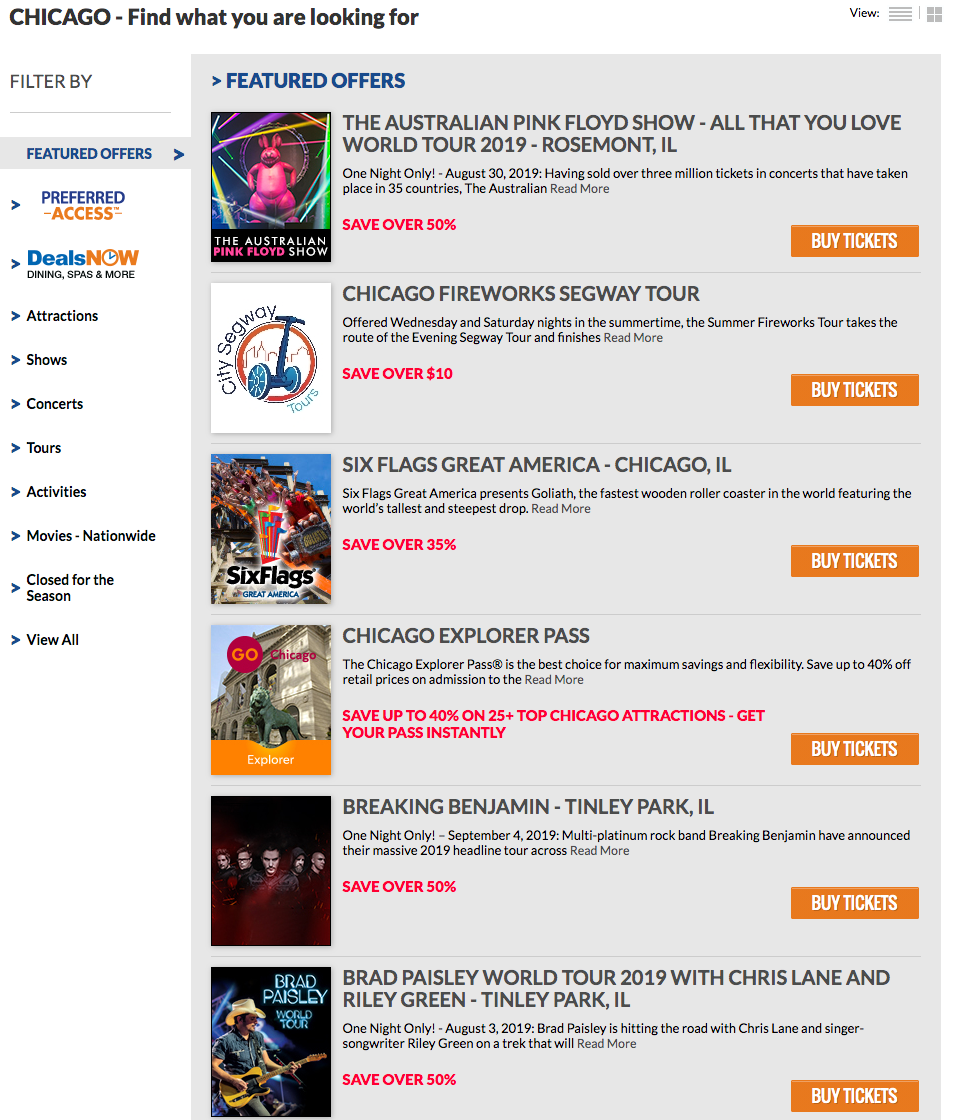### Detailed Caption for the Webpage Image Titled "Chicago - Find What You're Looking For"

The image presents a webpage titled "Chicago - Find What You're Looking For," featuring a variety of offers accompanied by images, detailed descriptions, and "Buy Ticket" buttons. Here's a detailed breakdown of each offer displayed:

1. **The Australian Pink Floyd Show**
   - **Tour Name:** All That You Love World Tour 2019
   - **Location:** Rosemont, Illinois
   - **Date:** August 30th, 2019 (One night only)
   - **Details:** This spectacular show has sold over 3 million tickets across concerts in 35 countries. 
   - **Offer:** Save over 50% on tickets.
   - **Buy Ticket:** Orange "Buy Ticket" button available.

2. **Chicago Fireworks Segway Tour**
   - **Description:** Available on Wednesday and Saturday nights throughout the summer. The summer fireworks tour incorporates the evening Segway tour route and concludes with a fireworks display.
   - **Offer:** Save over $10 on tickets.
   - **Buy Ticket:** Orange "Buy Ticket" button available.

3. **Six Flags Great America**
   - **Highlight:** Goliath, the fastest wooden roller coaster in the world, featuring the world's tallest and steepest drop.
   - **Location:** Chicago, Illinois
   - **Offer:** Save over 35% on tickets.
   - **Buy Ticket:** Orange "Buy Ticket" button available.

4. **Chicago Explorer Pass**
   - **Description:** The Chicago Explorer Pass, trademarked, is touted as the best choice for maximum savings and flexibility.
   - **Offer:** Save up to 40% off retail prices on admission for over 25 top Chicago attractions; get your pass instantly.
   - **Buy Ticket:** No specific button mentioned, but a "Read More" link is provided.

5. **Breaking Benjamin Concert**
   - **Location:** Tinley Park, Illinois
   - **Date:** September 4th, 2019 (One night only)
   - **Details:** The multi-platinum rock band Breaking Benjamin has announced their massive 2019 headline tour.
   - **Offer:** Save 50% on tickets.
   - **Buy Ticket:** Orange "Buy Ticket" button available.

6. **Brad Paisley World Tour 2019**
   - **Supporting Acts:** Chris Lane and Riley Green
   - **Location:** Tinley Park, Illinois
   - **Date:** August 3rd, 2019 (One night only)
   - **Details:** Brad Paisley is touring with Chris Lane and singer-songwriter Riley Green.
   - **Offer:** Save over 50% on tickets.
   - **Buy Ticket:** Orange "Buy Ticket" button available.

To the left of these listings, there is a "Featured Offer" section highlighting deals on dining, spas, attractions, shows, concerts, tours, activities, and movies, indicating that some options are closed for the season. There is also a "View All" link to explore more offers.

This caption provides a detailed description of the webpage’s content, highlighting various entertainment options available in Chicago along with exclusive ticket savings.